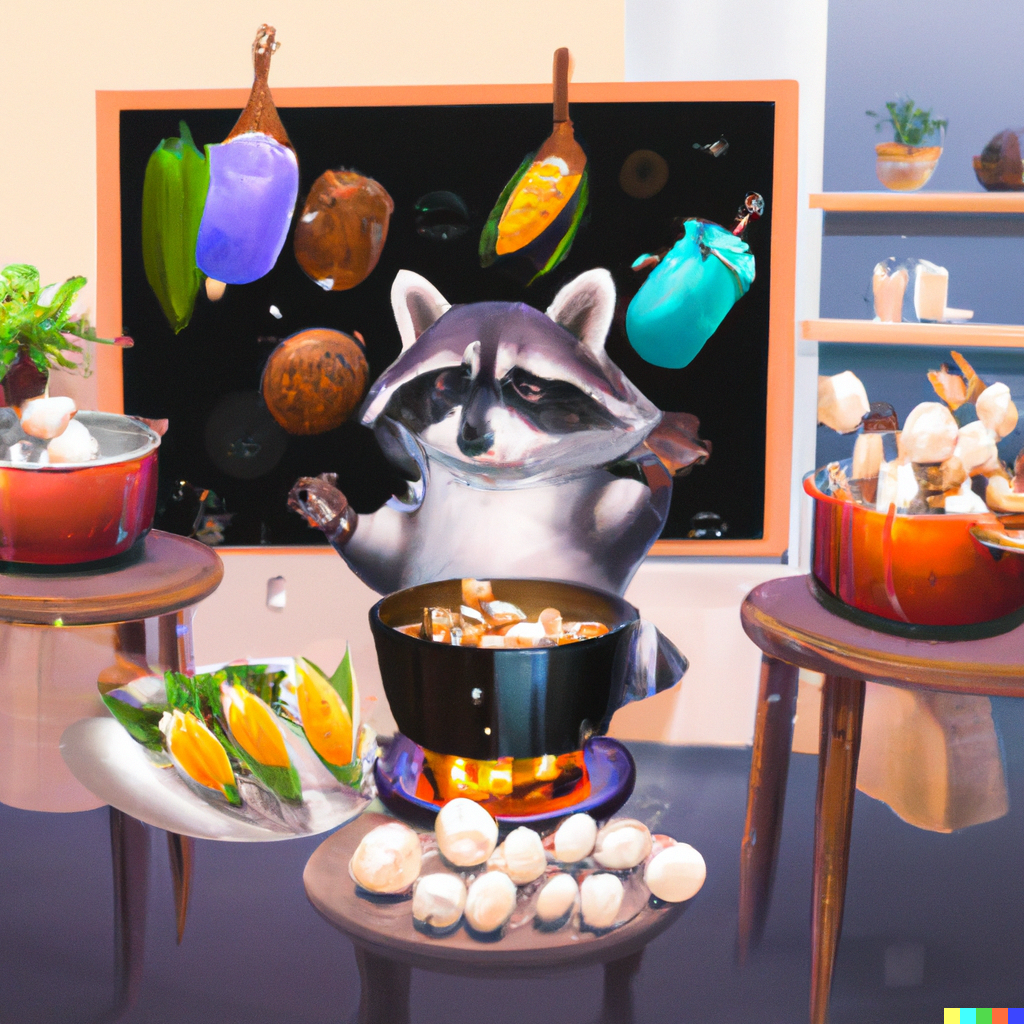This fanciful indoor graphic features a detailed scene of a raccoon standing and cooking in what appears to be a whimsical culinary setting, reminiscent of a cooking tutorial. The raccoon, depicted in shades of black and grey, stands behind a hot pot with visible heat emanating from it, cooking cubes of meat. The pot is positioned on a grey oval table that holds an assortment of boiled eggs. To the left floats a plate with three ears of corn, while on the right, a second oval wooden table supports a brown pot with pieces of cheese. 

In the background, two shelves on a blue wall hold various items: the top shelf with a bowl containing a green plant, and the middle shelf with two white containers. Behind the raccoon is a large blackboard with an orange border, illustrating several food items from left to right, including an ear of corn, a blue cutting board with a brown handle, a large nut, more corn, and a blue bag with an unidentified object protruding from it. 

Scattered throughout the scene are more culinary elements: an orange pot with white cheese pieces on another oval table, a grey-black vase with green plants, a color chart in the bottom right corner with shades of yellow, blue, turquoise, green, and orange, and various floating trays and containers. The raccoon's arms are held outward, adding to the impression that it is engaged in a cooking demonstration amidst this richly detailed, imaginative kitchen environment.